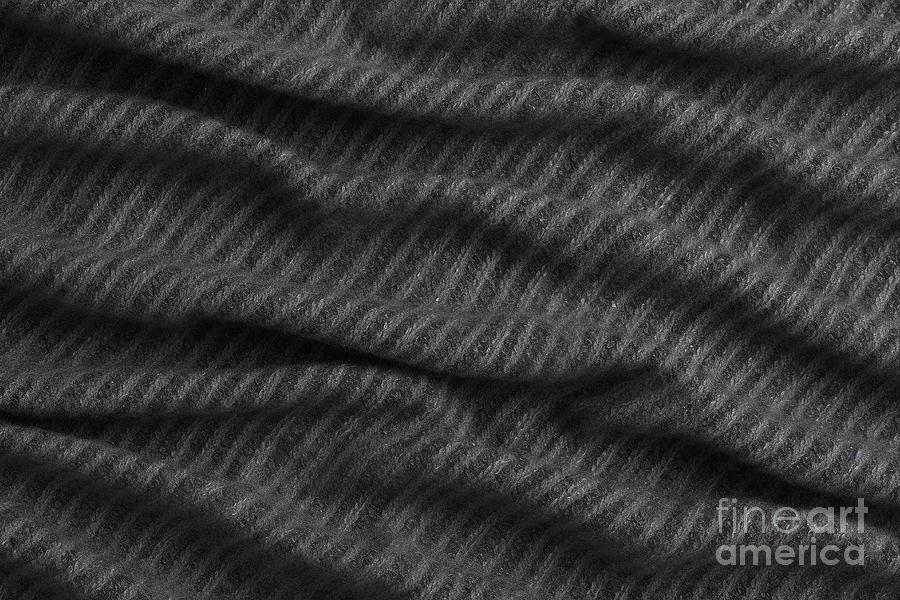This close-up photograph captures a semi-wrinkled piece of fabric, viewed from above. The fabric, potentially a towel or blanket, features a uniform pattern of alternating dark brownish-black and lighter grayish stripes. These diagonal stripes run from the bottom left to the top right, creating an undulating, textured landscape due to the slight bunching of the material. Despite its mundane appearance, the fabric fills the frame and is stamped with a Fine Art America watermark in the bottom right corner, suggesting its use in photo editing or as a texture reference. The fabric's versatile appearance and potential applications, from tapestry to carpet, highlight its intricate design that may be considered fine art by some.